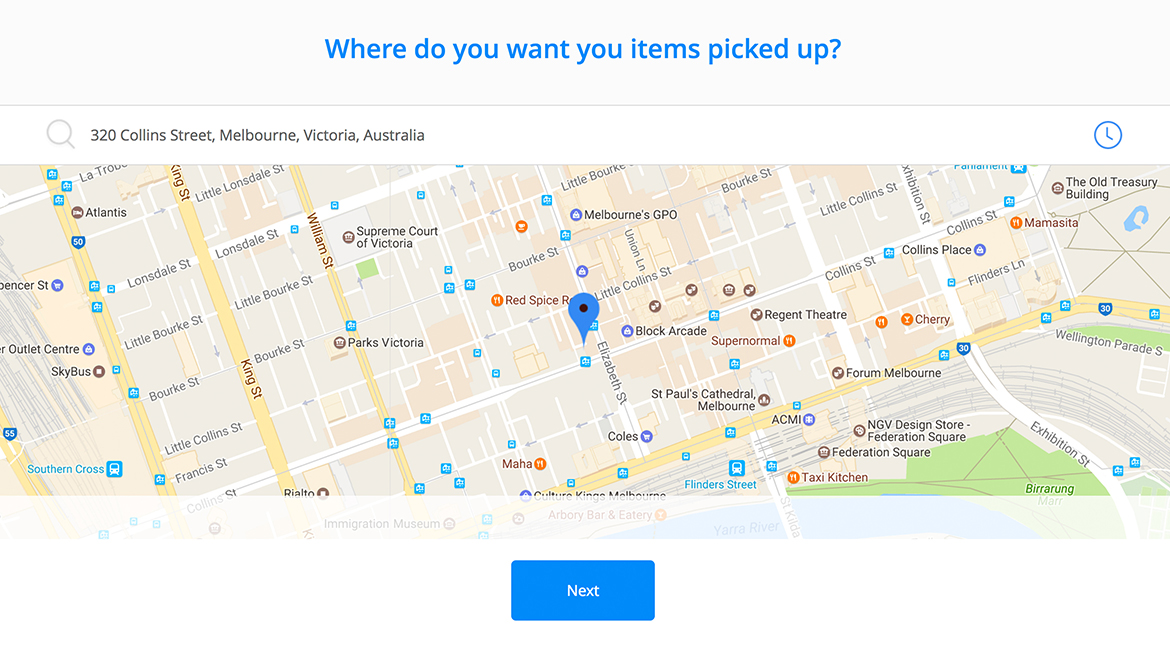This snapshot captures a website interface of what appears to be Google Maps, formatted within a horizontal rectangular frame. At the top of the image, a gradient area transitions from light blue to light gray, prominently featuring the text "Where do you want your items picked up?" in blue letters. Directly below this, a gray line spans the width of the frame, separating the top section from the main functional area.

Within the main area, a large white search bar stretches across the width. On the left side of this bar, the address "320 Collins Street, Melbourne, Victoria, Australia" is displayed. On the far right, a blue circle icon depicting a clock can be seen.

The central portion of the image showcases an interactive map. The map presents typical features such as streets marked in white, major highways in yellow, and green areas representing parks. Notable locations on the map include Williams Street, Parks Victoria, Exhibition Street, Little Collins Street, and St. Paul's Cathedral Melbourne, among others.

At the bottom of the image, a semi-translucent white strip overlays the lower portion of the map, and below this is a completely white area. In the center of this bottom section, there is a rectangular button with "Next" written in white letters.